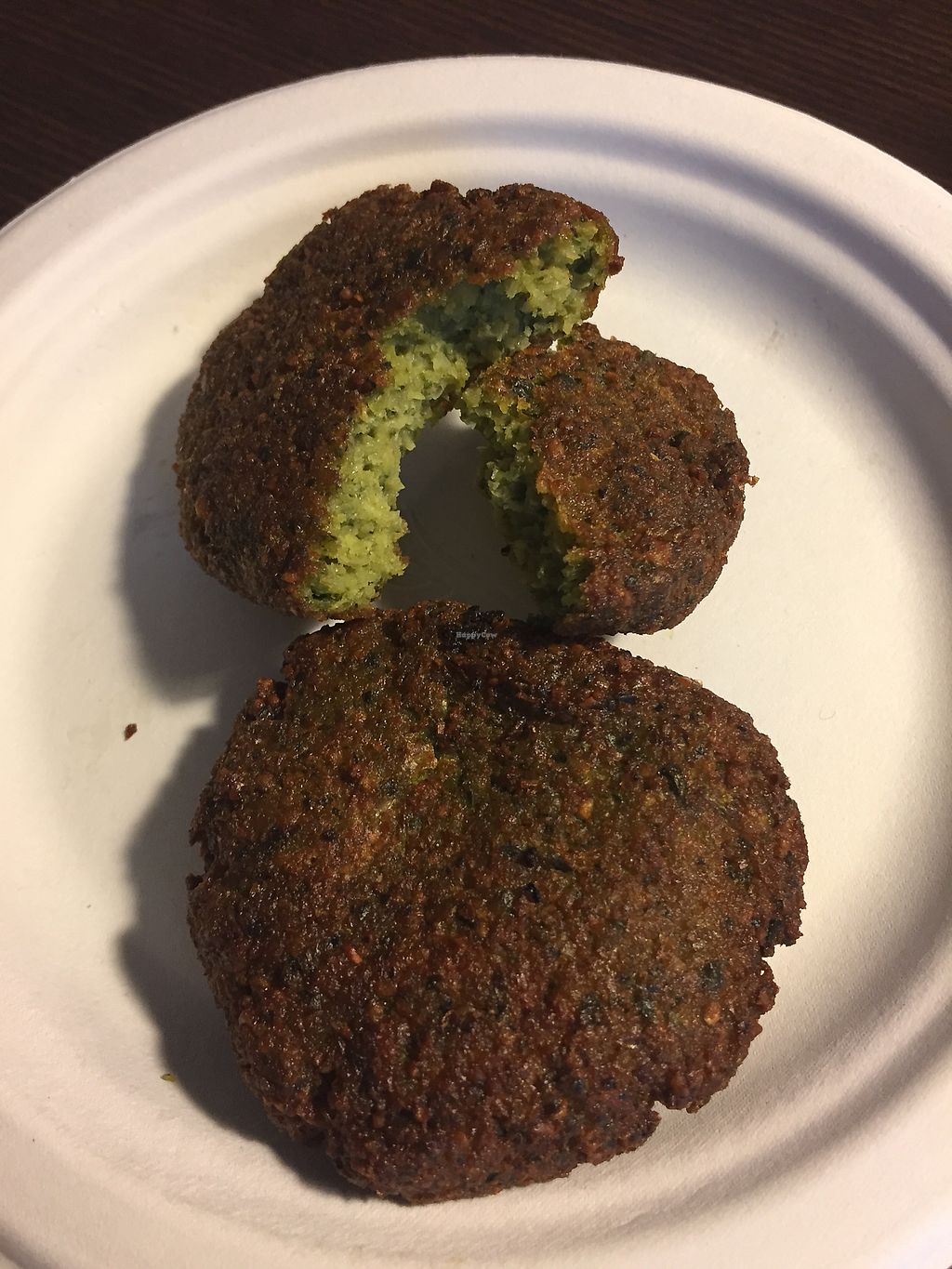This image features two fried falafel patties on a white paper plate against a black background. The patties are circular and dark brown on the outside, about the size of hockey pucks. The top falafel, partially broken with a bite taken out, reveals its vibrant yellowish-green interior with darker green specks, indicative of parsley. The second falafel patty, positioned slightly below and barely touching the first, remains intact. Both cast medium black shadows on their left sides due to the focused lighting. The plate is tightly cropped in the frame, with about 10% cut off from the right, left, and bottom, emphasizing the detailed texture and color contrast of the crispy, crumbly falafels.